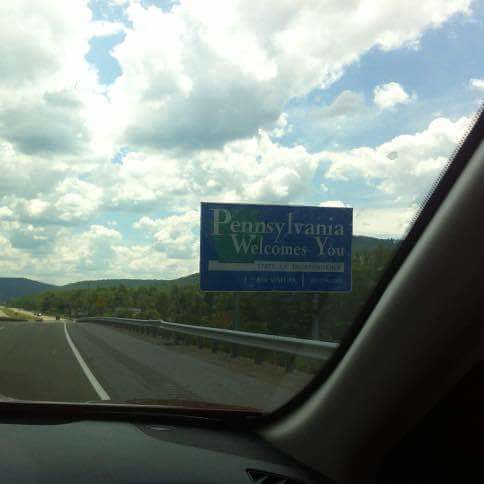The photograph captures the view from inside a gray car traveling along a highway, showing the landscape through the corner of the passenger side window. Prominently visible is a large rectangular blue sign with white letters that reads "Pennsylvania Welcomes You," indicating that the vehicle is entering Pennsylvania. The highway is lined with a guardrail on the right side, and there's a white line marking the road edge alongside the corrugated area designed to vibrate the car if hit. Off in the distance, the road is dotted with cars heading along the same route, disappearing into a serene landscape of rolling hills and lush pine trees. The horizon reveals a striking backdrop of mountains reaching up towards a vast blue sky, adorned with billowing, fluffy clouds illuminated by the bright sunlight piercing through. The serene scene outside contrasts with the functional details inside the car, such as the visible heater vents at the bottom of the window frame.